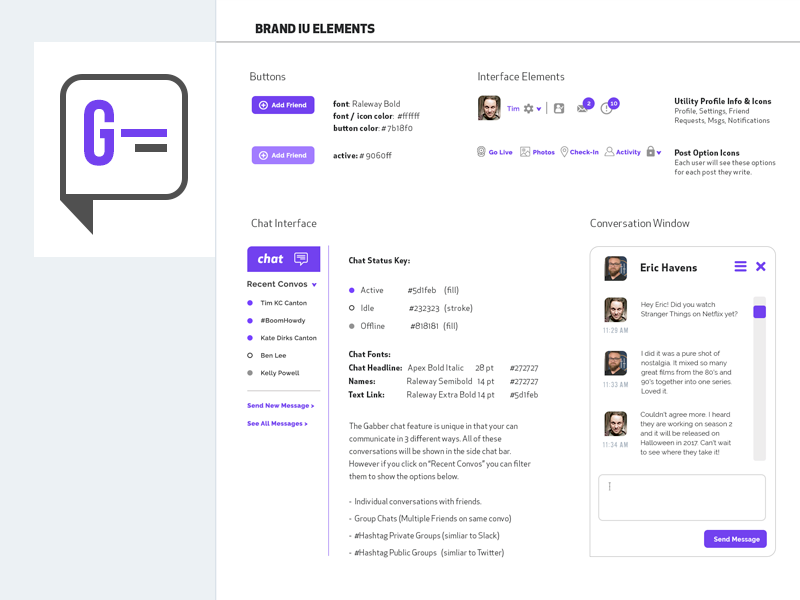The image displays a comprehensive UI reference page, featuring a variety of elements used in the design. In the top left corner, there's a large letter "G". Directly to the right, the title "Brand UI Elements" is prominently displayed. The layout is meticulously organized, serving as an intricate guide to different interface components.

In the "Buttons" section, there is an "Add Friend" button alongside a grayed-out version of the same button, indicating its inactive state. 

The "Interface Elements" section includes icons and text for various functions, such as unread messages and settings.

Below this, a "Chat Interface" section outlines the features available in the chat application, including information about user status (active, idle, or offline). Each status indicator has a corresponding code for easy reference.

Positioned in the bottom right of the page, there's a "Conversation Window" showcasing a sample chat between two individuals, Eric Havens and another person. The conversation highlights a casual discussion about watching the TV show "Stranger Things" on Netflix, with one person expressing that it delivered a strong sense of nostalgia.

Overall, the page serves as a detailed map of the UI elements, effectively illustrating the various components and their designated uses.